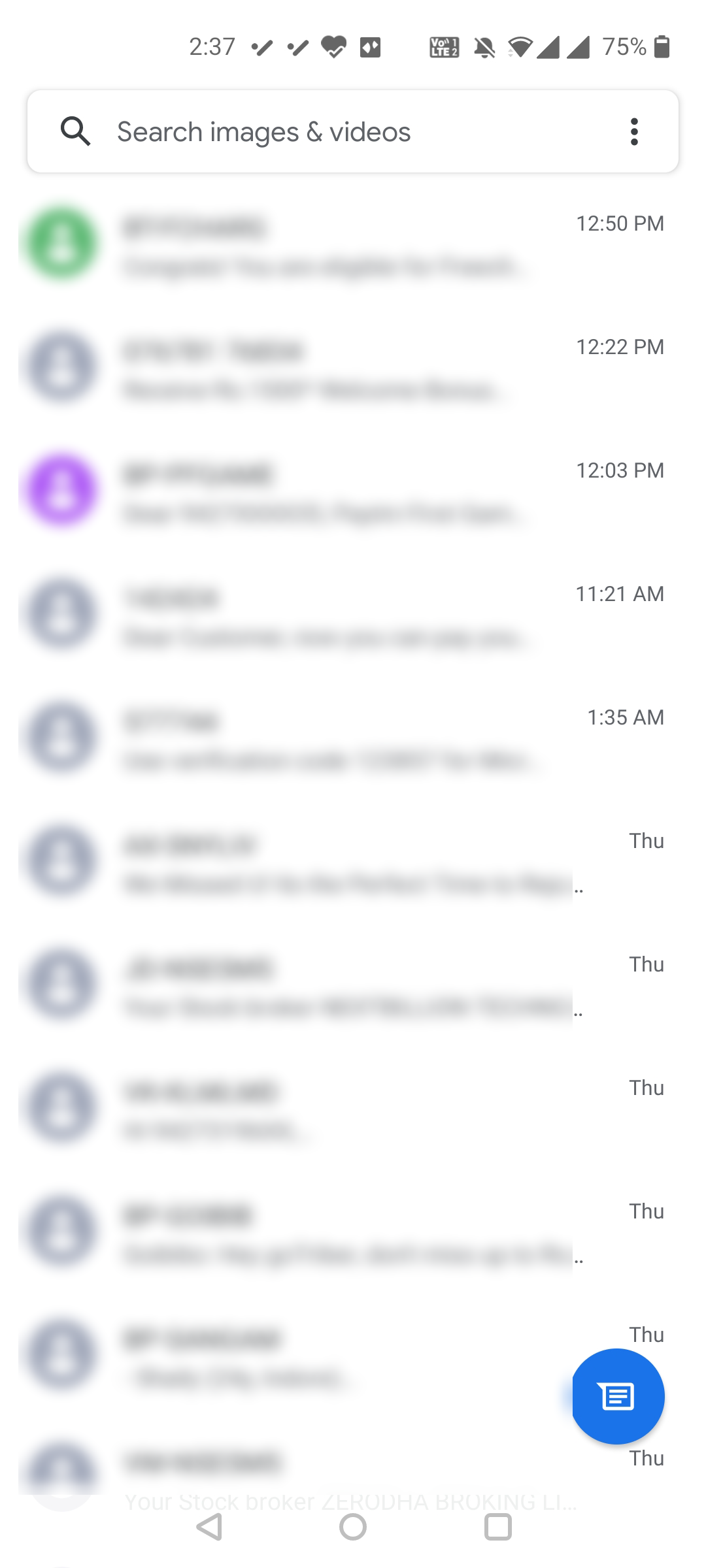The image depicts a cell phone screen with a blurred app interface. The phone’s information bar at the top shows a battery level at 75%, muted notifications, and an active Wi-Fi connection. The current time displayed is 2:37. The app, whose identity is uncertain due to blurring, features a search box at the very top labeled "Search images and videos", suggesting that the user might be searching through their personal media library.

However, all images and search results below this box are intentionally blurred out for privacy. Despite this blurring, the timing of the search results is visible, showing entries listed at 12:50 p.m., 12:22 p.m., 12:03 p.m., 11:21 a.m., and 1:35 a.m. Following these times, subsequent entries are marked simply with "Thursday", implying they were searched the previous day.

The presence of notifications, possibly from a health app and Patreon, further contextualizes the user's activity. Despite privacy measures taken on the content, the image has been posted online.